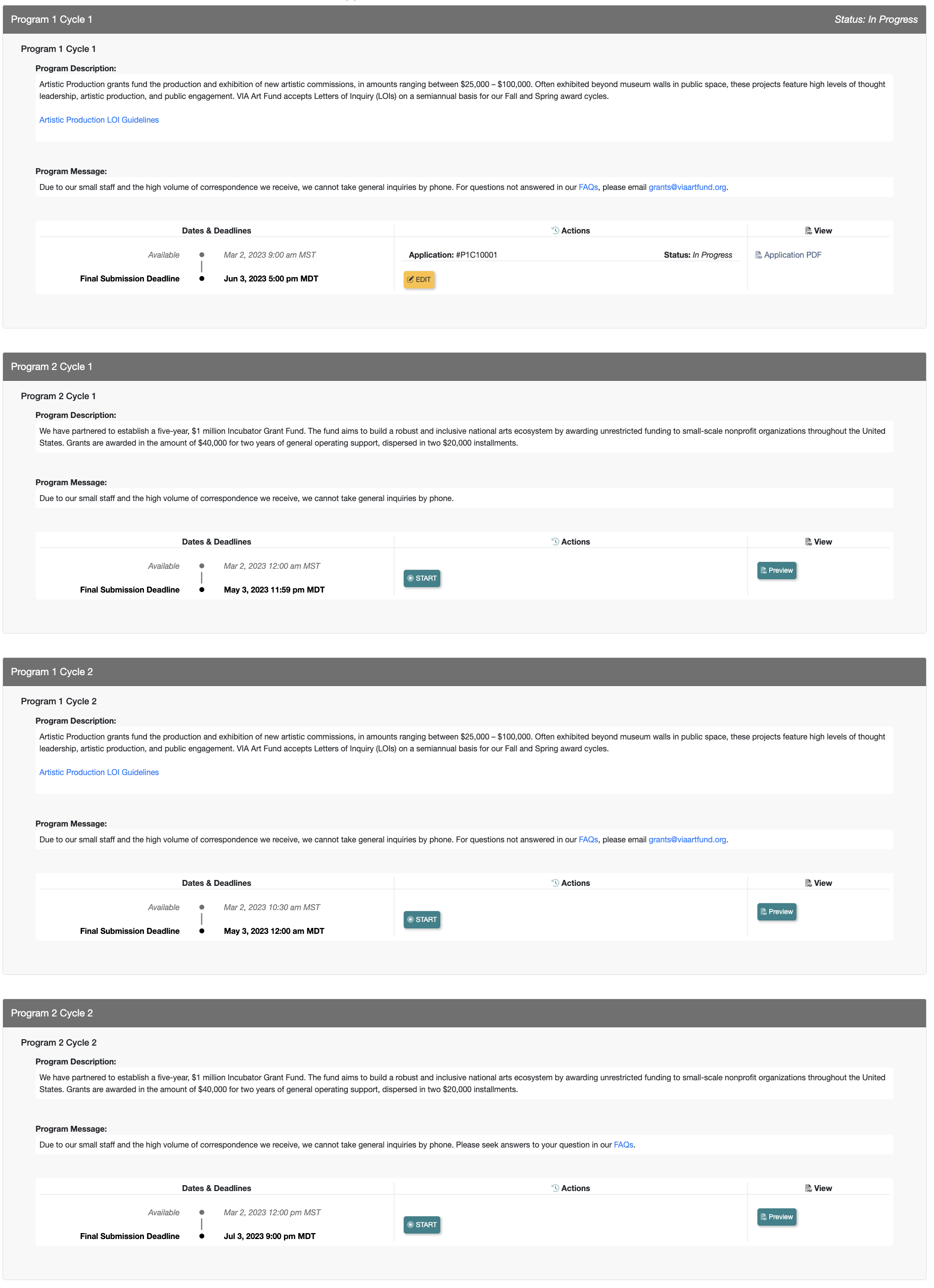The top edge of the website features a gray bar with white text that reads "Program 1, Cycle 1." On the right side, there are the sections labeled "Status" and "Progress." Below this is a white background with black text that outlines the details of "Program 1, Cycle 1, Program Description." This section explains that the Artistic Production Grants fund the production and exhibition of new artistic commissions, awarding amounts between $25,000 and $100,000. These projects, often showcased both within and beyond museum walls in public spaces, emphasize high levels of thought leadership, artistic production, and public engagement. The WIA Art Fund accepts letters of inquiry (LOIs) semi-annually for their fall and spring award cycles. 

A clickable link titled "Artistic Production LOI Guidelines" is displayed in blue below this description. Following this, there is another section titled "Program Message" against a gray background with white rectangles for text. It states that due to the small staff size and high volume of correspondence, general inquiries cannot be taken by phone. For questions not covered in the FAQs, which are linked in blue, individuals are encouraged to email grants@wiaartfund.org.